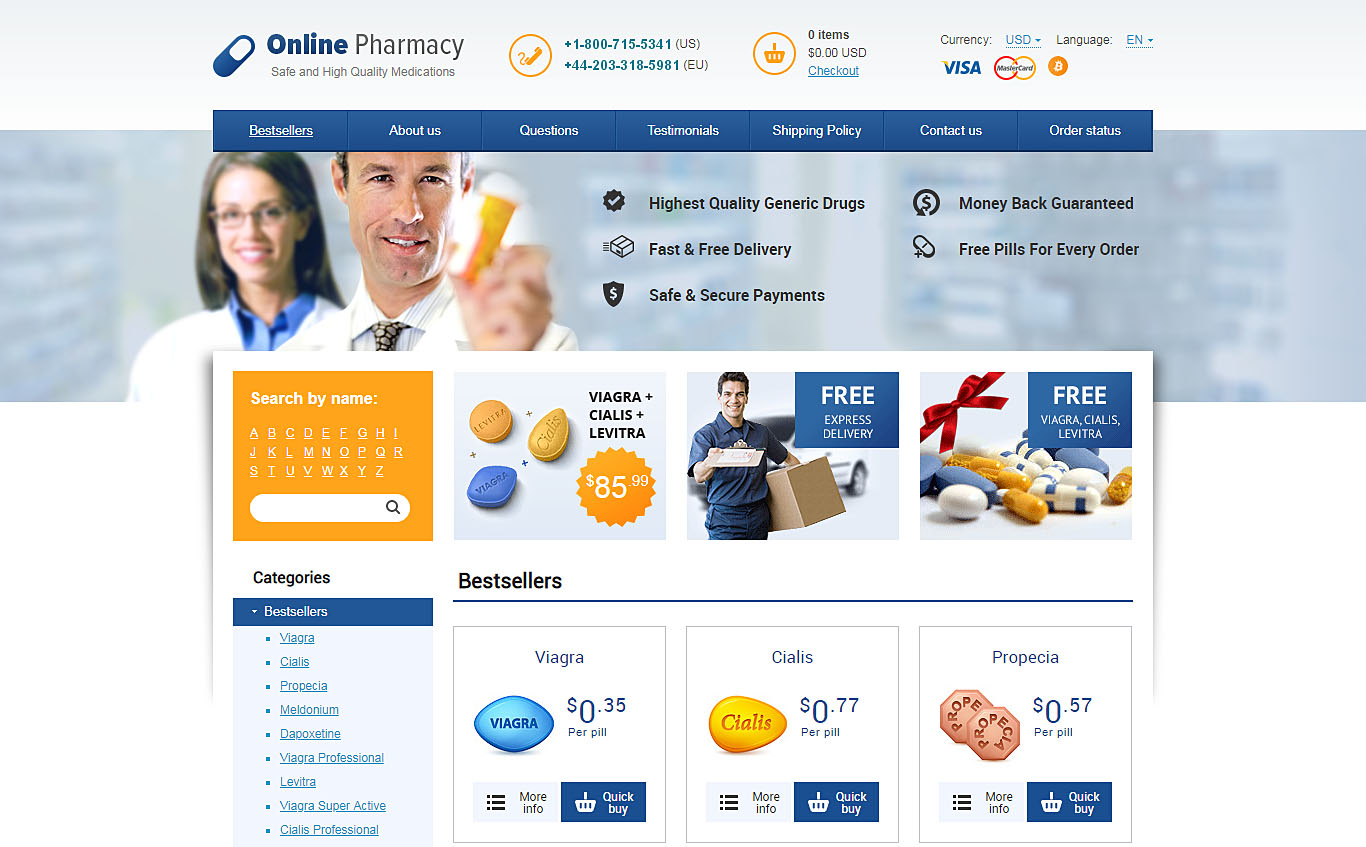### Detailed Caption for Online Pharmacy Website Image

The website header displays "Online Pharmacy" in a bold, prominent font. In the upper left-hand corner, a blue and white pill logo signifies the brand. Adjacent to the logo, there's a circular icon featuring an orange phone symbol. To the right of this icon, contact numbers are listed in an aquamarine hue: "1-800-715-5341-US" and "44-203-318-5981-EU".

Next to the contact numbers, there is a shopping cart icon displaying "0 items" with a total of "$0.00 USD" and a "Checkout" button. The currency is currently set to USD. Payment options are indicated by Visa, MasterCard, and Bitcoin icons. A language selection option, denoted by "Yen for English," is also visible.

Below this header, a navigation bar presents various sections: "Best Sellers," "About Us," "Questions," "Testimonials," "Shipping Policy," "Contact Us," and "Order Status," each styled with blue buttons and white text, separated by small dividers.

The main content features an image of a man and a woman dressed as doctors. Both appear to have European heritage and brown hair. The man is offering an orange pill bottle towards the viewer. This section promotes "Highest Quality Generic Drugs," "Money Back Guaranteed," "Fast and Free Delivery," "Free Pills for Every Order," and "Safe and Secure Payments."

Further down, there is an "A-Z" search section with a white search bar against an orange background. Adjacent to it, a promotional box advertises "Viagra, Cialis, Levitra" for $85.99, featuring images of the pills and an orange price tag. Another box offers "Free Express Delivery," showcasing a delivery man with brown hair in a blue shirt, holding a clipboard.

Next to this, there is a banner for "Free Viagra, Cialis, and Levitra," pictured with orange, white, and blue pills tied with a red bow. 

On the left side, the website categorizes products under "Best Sellers," "Viagra," "Cialis," "Propecia," "Meldonium," and "Diprogextine." A blue line serves as a divider, and underneath, three product boxes are displayed: "Viagra" ($0.35/pill, blue), "Cialis" ($0.77/pill, yellow), and "Propecia" ($0.57/pill, red), each with "Quick Buy" and "More Info" buttons.

This image captures the detailed layout and offerings of an online pharmacy website, highlighting its structure, contact information, payment options, and promotional deals.